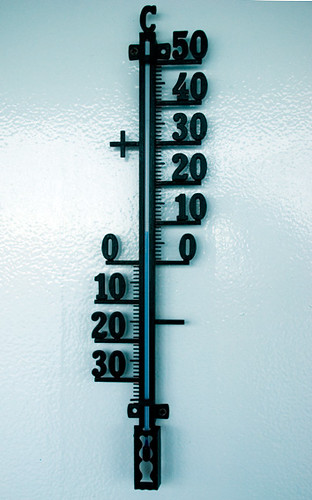The image appears to depict a large, vertical thermometer-like instrument mounted on a shiny, light blue wall. The wall is highly reflective, creating a gleaming surface that adds to the visual distinction of the instrument. At the top of this vertical structure, there is a black, capital "C" prominently displayed. The structure itself is a long, slender black metal strip running from the top to the bottom.

On the right side of the strip, there are numerical markings starting with "0" at the bottom and ascending in increments of ten—10, 20, 30, 40 up to 50. Each number is accompanied by a horizontal line just below it, with smaller tick marks to its left indicating finer measurements.

Similarly, on the left side of the strip, there are corresponding numbers 0, 10, 20, 30, 40, and 50. These numbers also have horizontal lines beneath them, and each mark aligns with the corresponding number on the right side.

In the middle of this instrument, there appears to be a light blue liquid that rises vertically up the scale, almost reaching the 10 mark on the right side. At the bottom of the instrument, there are two black horizontal bars separated by a small gap, which might signify the base or the starting point of the measurement.

Overall, the resemblance to a thermometer, specifically a centigrade one, suggests that this instrument is used for measuring temperature.